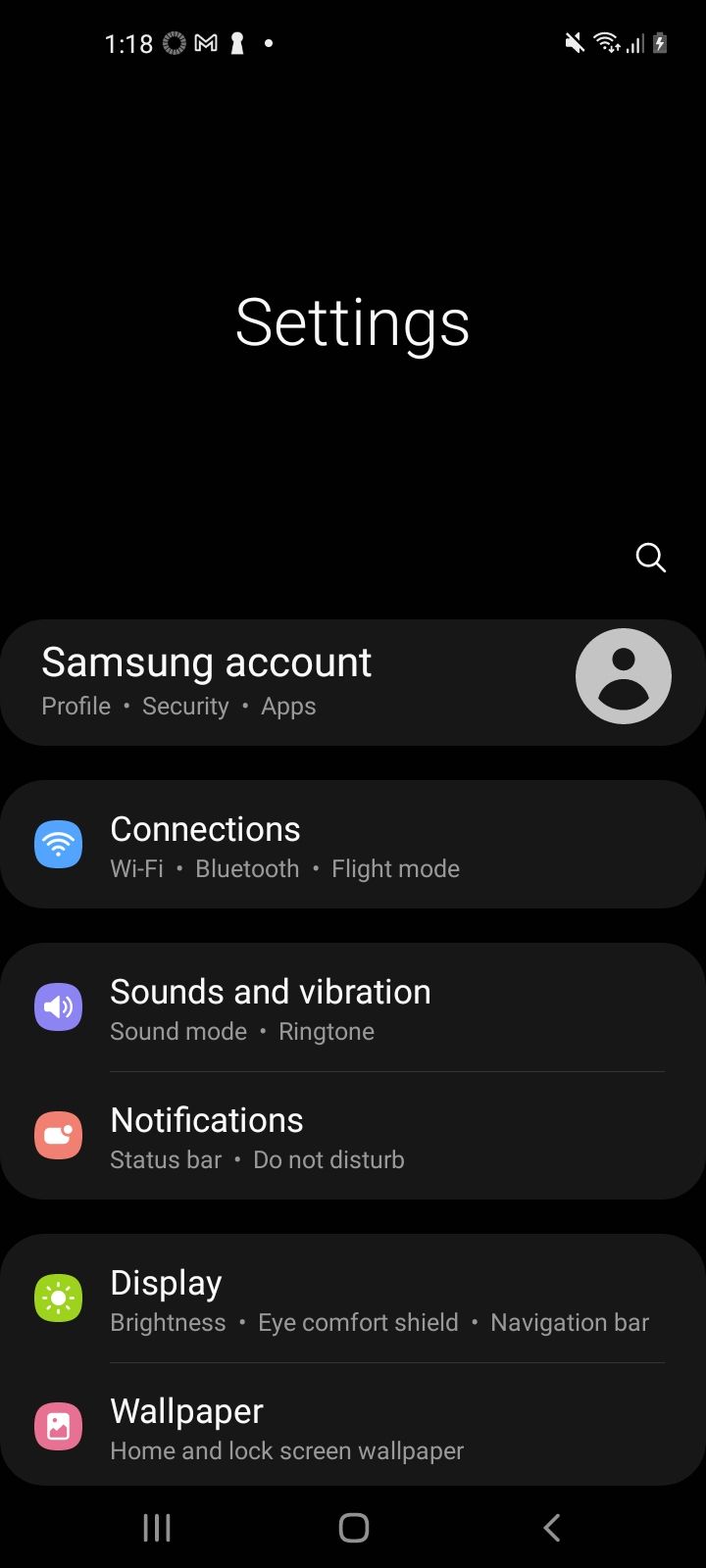Screenshot of a Samsung phone displaying the Settings menu against a black background. The settings text is in white, and a picture icon appears on the right without a photo. The main categories listed are:

- **Profile, Security, Apps:** Indicates user account options and security settings. 
- **Connections:** Shown in blue, detailing "WiFi," "Bluetooth," and an active "Flight mode."
- **Sounds and Vibration:** Noted by a purple icon resembling a side ringer bell, with options for Sound mode and ringtone.
- **Notifications:** Displayed with an orange background and a white bubble, featuring options for Status bar and Do Not Disturb.
- **Display:** Highlighted in green with a sun icon, covering settings like brightness, eye comfort shield, and navigation bar.
- **Wallpaper:** Displayed in pink, addressing Home and Lock screen wallpapers.

At the screen’s bottom right, the status bar shows the time as 1:18, indicates an active WiFi connection with three bars, and a battery icon suggesting a good charge level.